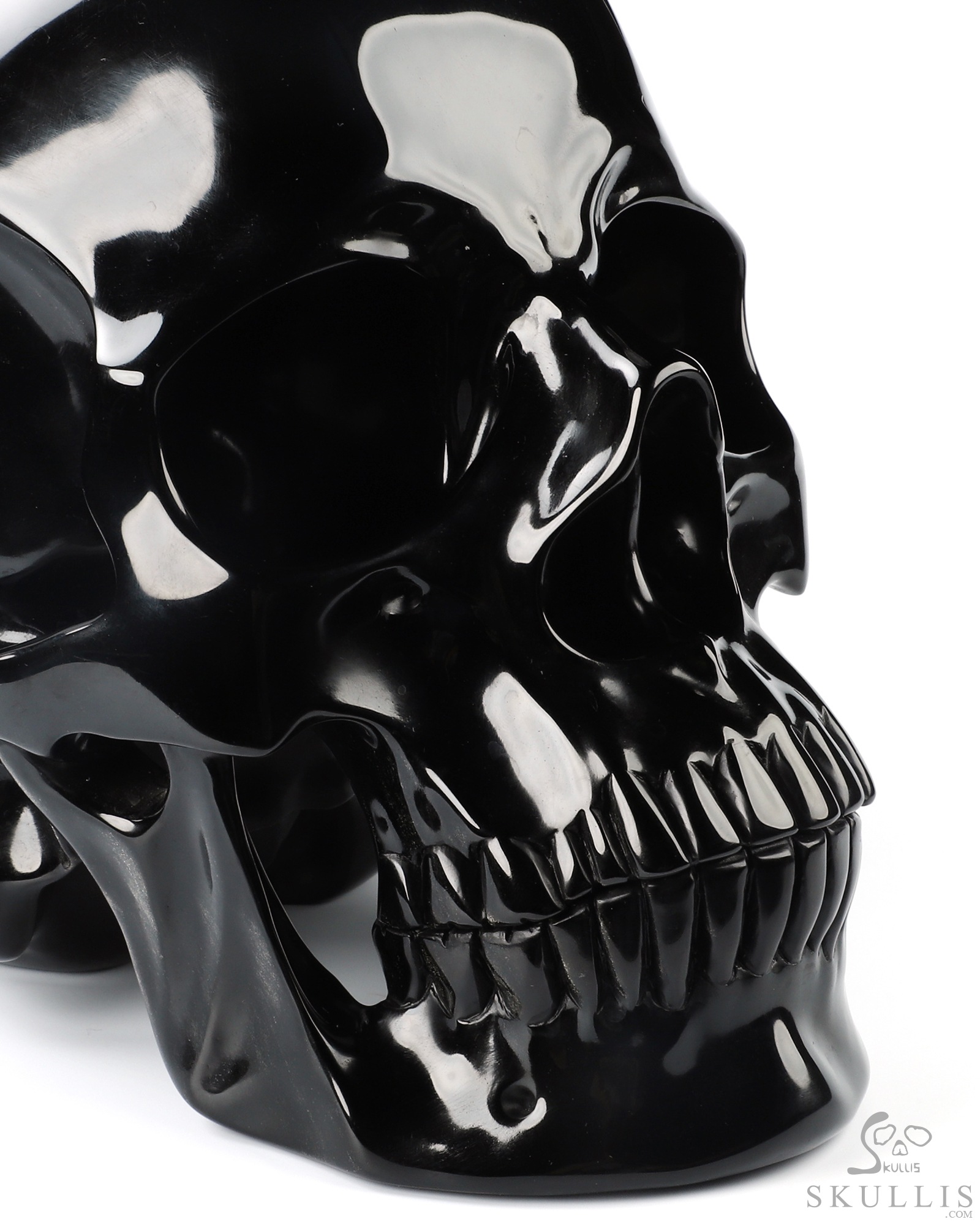The image is a striking promotional photograph for a website, skullis.com, indicated by the watermark in the bottom right corner. The text "skullis.com" is presented in gray, with a logo above that features an 'S' with eyes represented by two circles, a nose as a triangle, and the continuation of "K-U-L-L-I-S" forming the mouth to spell out "SKULLIS." The main focus of the image is a shiny, black metallic human-like skull, set against a stark white background and resting on a white table. The skull has an intense, intimidating appearance, with pronounced eye cavities, a nasal opening, and visible teeth. Its surface appears to gleam under the light, giving it a highly polished, almost plastic-like finish. The skull is tilted at an angle, cutting off a portion of its structure from the frame, adding to the dramatic effect of the composition.